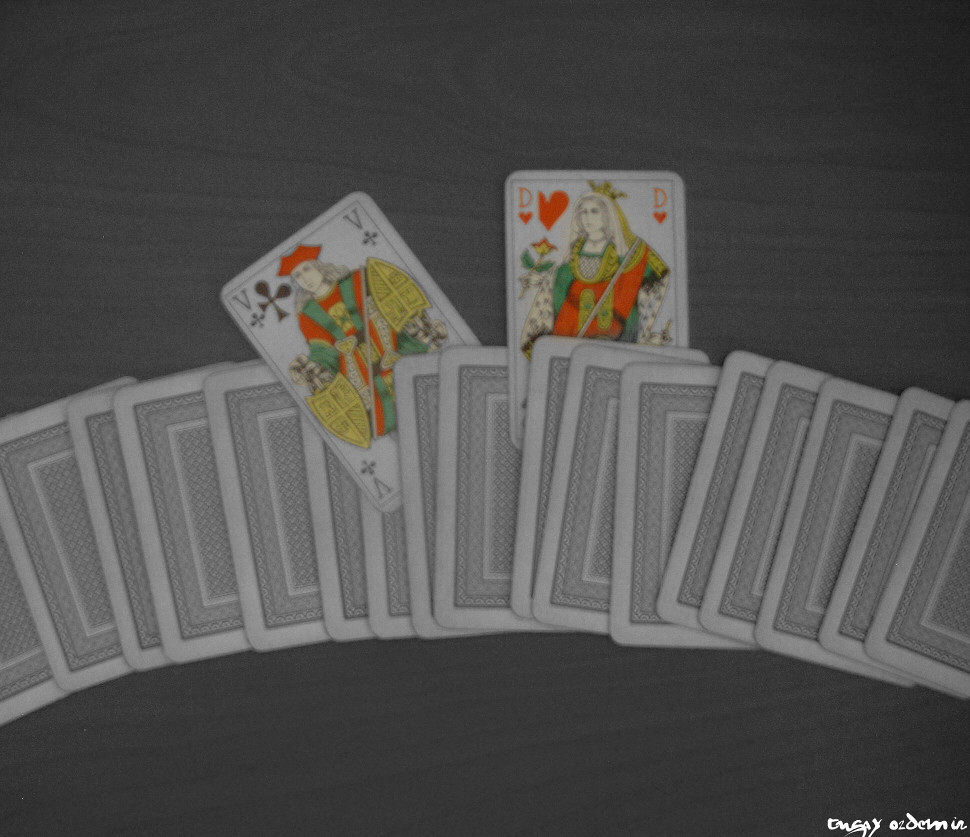A spread of playing cards is artfully laid out on a rustic gray wooden table. All cards are facedown, displaying their white borders adorned with some black detailing. Intriguingly, two cards have been flipped over to reveal their faces. One card features a king, denoted by the letter "V" instead of the traditional "K," and the other features a queen, marked with a "D" instead of the usual "Q." Both figures are dressed in vibrant red-green outfits, adding a whimsical touch to the scene. The king's card is adorned with yellow shields, enhancing his regality. The substitution of "V" and "D" for "K" and "Q" invites speculation about their significance, perhaps hinting at characters named Valaldi and Dresden. The overall setting suggests an air of mystery and prompts reflection on potential stories behind these captivating cards.